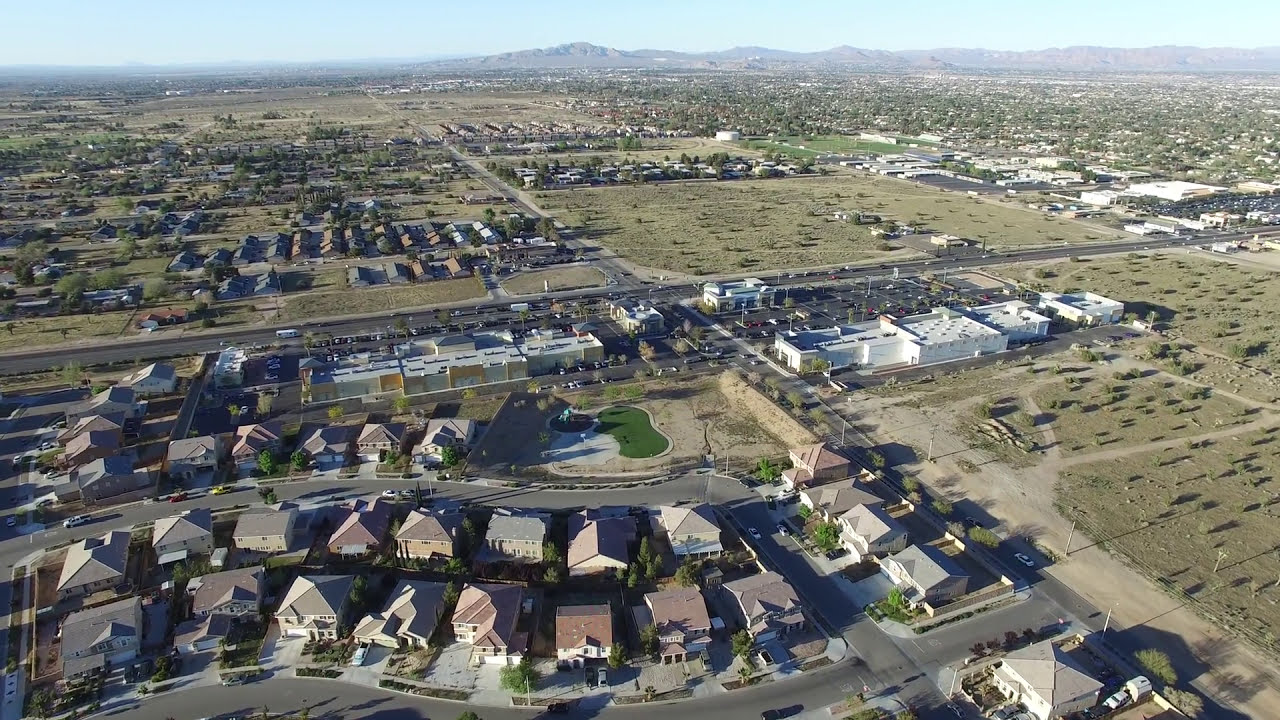This aerial color photograph, taken from a bird's-eye view, captures a diverse landscape in landscape orientation. At the bottom left corner, rows of similar-looking residential houses, tightly packed with small trees in their yards, are visible. Towards the bottom right, a road stretches diagonally from the bottom right corner towards the center, intersecting with another road that extends from the left side towards the top right of the image. To the right of the first road, there are patches of bare ground and green pastures, contrasting with the structures on the left. As the eye moves further up, a shopping center with a notable parking lot appears near the center of the image. Scattered buildings and small trees are noticeable throughout. The horizon is dominated by a distant mountain range that is most visible in the middle and right parts of the image, with a thin strip of blue sky stretching across the top. The color palette includes gray, brown, green, white, yellow, orange, red, and blue, reflecting the diversity of objects and natural elements. The overall scene is flat with mountains in the distance, captured in the middle of the day.